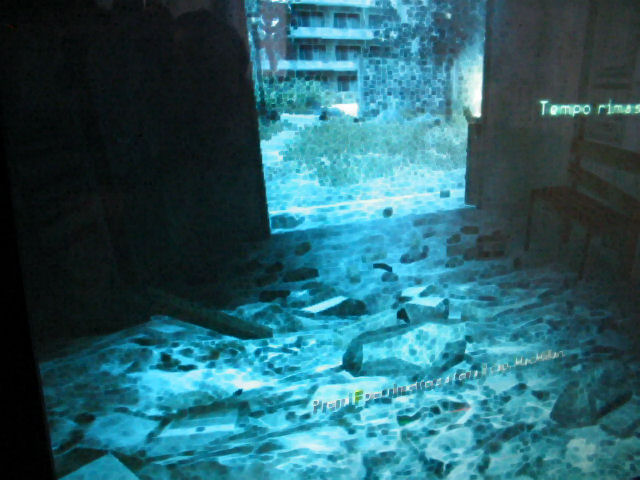The image portrays a desolate, bluish-tinted scene inside a dimly lit room with a floor covered in white and gray cobblestones or rubble. The view is directed towards an open doorway, through which an overgrown, neglected exterior can be observed. Outside, the scene is dominated by an abandoned apartment complex across the way, featuring a brick building with three floors, numerous rectangular windows, and possibly some doors. Weeds and overgrowth are visible along the walls and a nearby fence, highlighting the area’s long-term abandonment. The image quality is notably low, with a blurred, off-color blue tint that distorts the true colors. Superimposed text appears on the top right corner with words looking like "tempo RIMAS," seemingly burned onto the image, while illegible dialogue-like text can be found near the bottom, suggesting that this may be a still from a low-quality video game or digital art piece set in a war-torn environment.